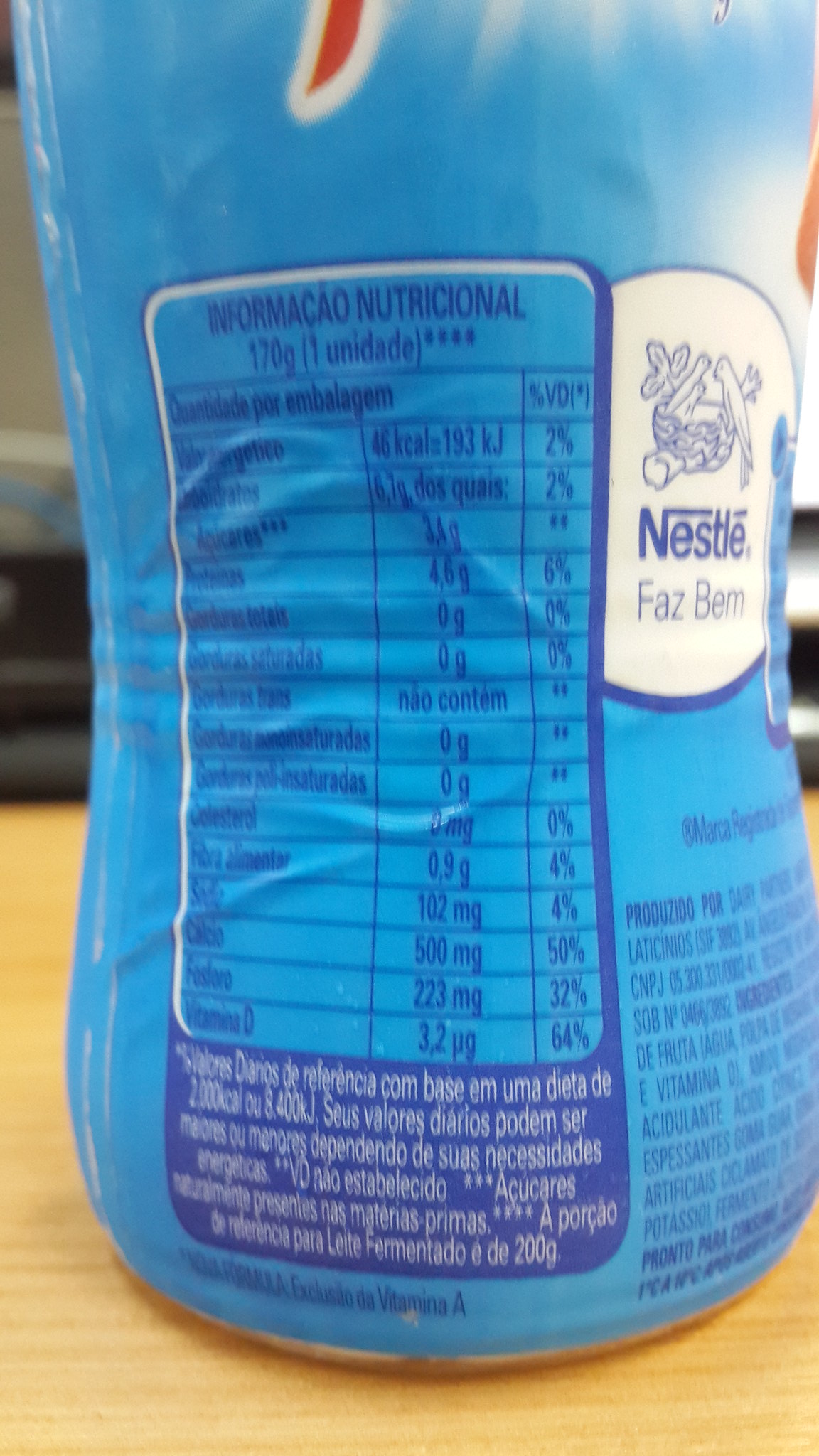This is a high-resolution photograph of the back label of a product bottle placed on a textured wooden surface, which is a light beige color with prominent dark grains running through it. The bottle, which occupies much of the frame and is positioned centrally, features a blue label that outlines the product’s nutritional information, primarily in Portuguese. The visible section of the bottle is the bottom half, making the nutrition facts the focal point of the image. 

Highlighted on the label is the phrase "Informação Nutricional," which confirms the language as Portuguese. Below this heading, it lists "170g" with several asterisks next to it, potentially denoting footnotes or additional information. The nutrition facts table is structured into three columns and approximately fifteen rows, providing detailed information on the product's nutritional values. 

Additionally, beneath this table, there is a paragraph of text in Portuguese, which seems to further elaborate on the nutritional information or provide some regulatory details.

On the right side of the label, there is a distinctive white shape featuring the recognizable Nestlé logo with the text "Nestlé" below it, followed by the words "Faz Bem." Below this logo, there is an area of blue text on the light blue label, which likely lists the ingredients of the product. This ingredient list is comprehensive, containing numerous components written in Portuguese. 

Overall, the photo captures the intricate details of the label, allowing viewers to glimpse both the nutritional information and the branding elements of the product. The background hints at an object behind the bottle, partially obscured and unidentified, adding depth to the composition.